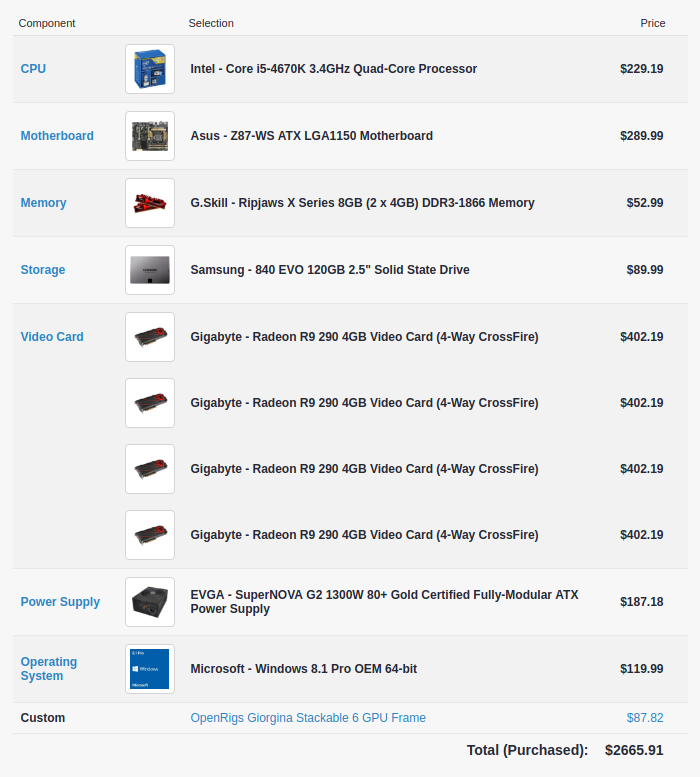A customer is shopping for high-performance computer components. The selected items include an Intel Core Quad Processor priced at $229.19 and an Asus Motherboard for $289.99. Memory requirements are met with G.Skill Ripjaws X-Series 8GB 1866MHz modules at an astonishing $5,299. For storage, a Samsung 840 Evo 120GB 2.5" Solid State Drive is priced at $89. Additionally, a Gigabyte Radeon R9 290 4GB Video Card is listed at $402.19. Power needs are covered by an EVGA SuperNova G2 Gold-Certified Fully Modular ATX Power Supply for $187.18. The system operates on Microsoft Windows 8.1 Pro 64-bit, with a license costing $119. Finally, a custom OpenRig's Georgiana Stack of 06 GPU frame is included for $87. The total cost for the selected components amounts to $2,665.91, making it a significant investment for a high-end build.